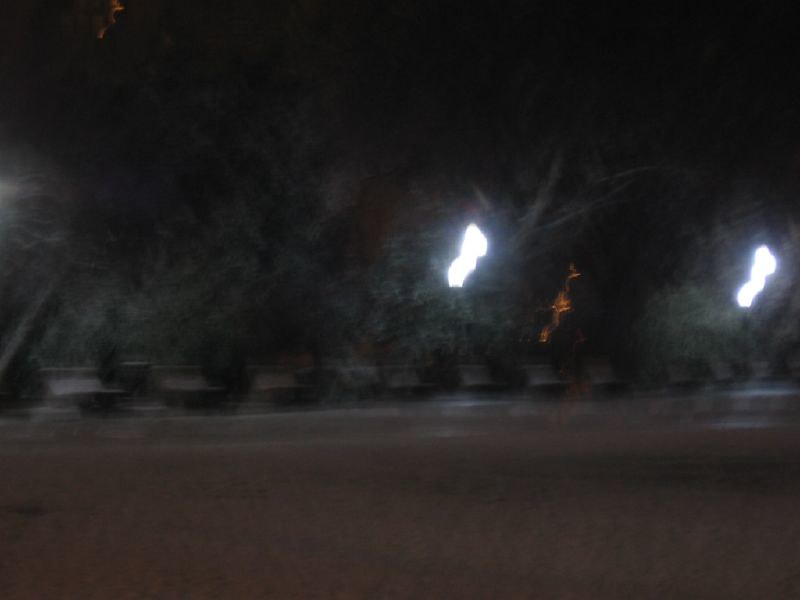In this blurry night scene set outdoors, the foreground showcases a brown, paved area. Toward the end of this paved section, several concrete seats or boxes with concave shapes and edges on both sides are arranged, forming a sort of perimeter around the area. In the background, blurry trees are faintly visible, adorned with scattered lights. Specifically, one bright light is positioned on the right-hand side, while another light can be seen toward the center of the trees. Just below the central light and slightly to the right, there is a distinctive, orange glow resembling a flame. The sky above is predominantly black, with a subtle hint of orange in the upper left corner, adding to the overall dark and mysterious ambiance.